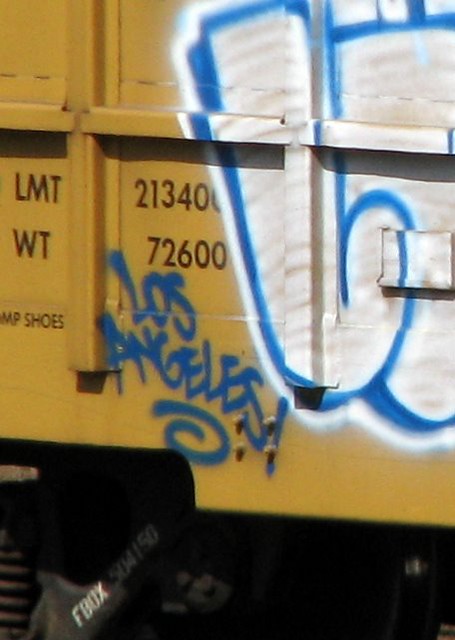This photograph captures a close-up of the side of a mustard-yellow boxcar, focusing on the lower portion of the rail car. Prominent graffiti dominates the upper right section, featuring large white bubble letters outlined in a vibrant blue hue. Though the text isn't fully legible, the first letter appears to be an 'L.' Adjacent to this graffiti, written in stylish slanted blue script, is the word "Los Angeles" with an exclamation mark and a decorative spiral beneath it. Additional details include several mechanical parts visible at the bottom, such as springs, a wheel, and an axle marked "FBOX504150" at an upward slant. The car itself bears imprinted text, with numbers and codes like "LMT 213400," "WT 72600," and the word "SHOES." The intricate blend of colors, tag lines, and train details create a striking and rich visual narrative.